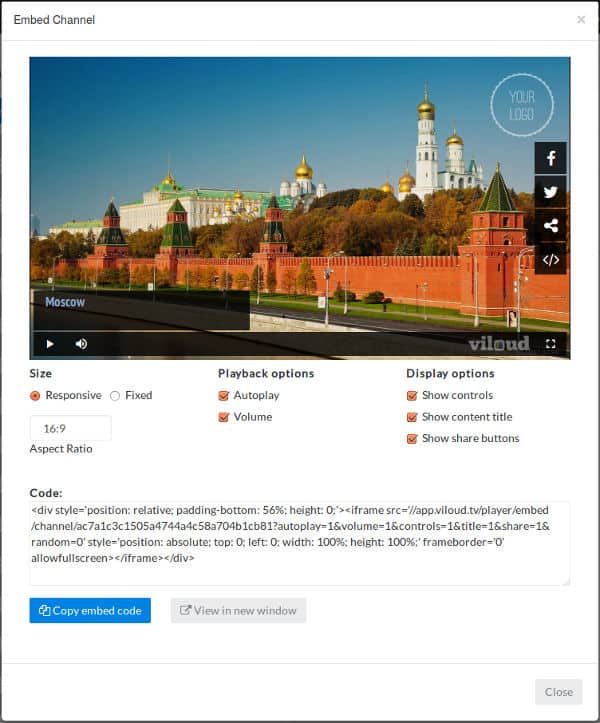The web page features a central image framed by a thin black line, set against a white background. At the top left corner of the page, there's the label "Embedded Channel." Below this label, a captivating image of a cityscape showcases an array of large white towers adorned with golden domes. A prominent white building with golden domes and a green roof stands out in the background. A brick wall and rows of trees line the front of these structures, accompanied by a street with streetlights visible.

To the right of the cityscape image, social media icons are displayed vertically: a Facebook logo, followed by a Twitter logo, a share icon, and arrows pointing left and right, respectively. At the bottom left corner of the image, a play button is situated, while a sound button is located at the bottom right, labeled "Bill Loud," alongside a full-screen option.

On the left side below the play button, various settings are neatly arranged against the white background. The "Size" option is followed by "Playback Options" and "Display Options." Next to "Playback Options," circles indicate "Responsive" and "Fixed," with "Responsive" selected in orange. Below "Playback Options" are "Audio Play" and "Volume," both highlighted in orange squares. Under "Display Options," checkboxes for "Show Control," "Show Content Title," and "Show Share Buttons" are all marked in orange.

Further down, the section labeled "Code" contains several URL links. At the bottom left, there's a blue "Copy Embed Code" button, adjacent to a grey "View in Windows" button. In the bottom right corner, a grey button with black letters serves as the "Close" button.